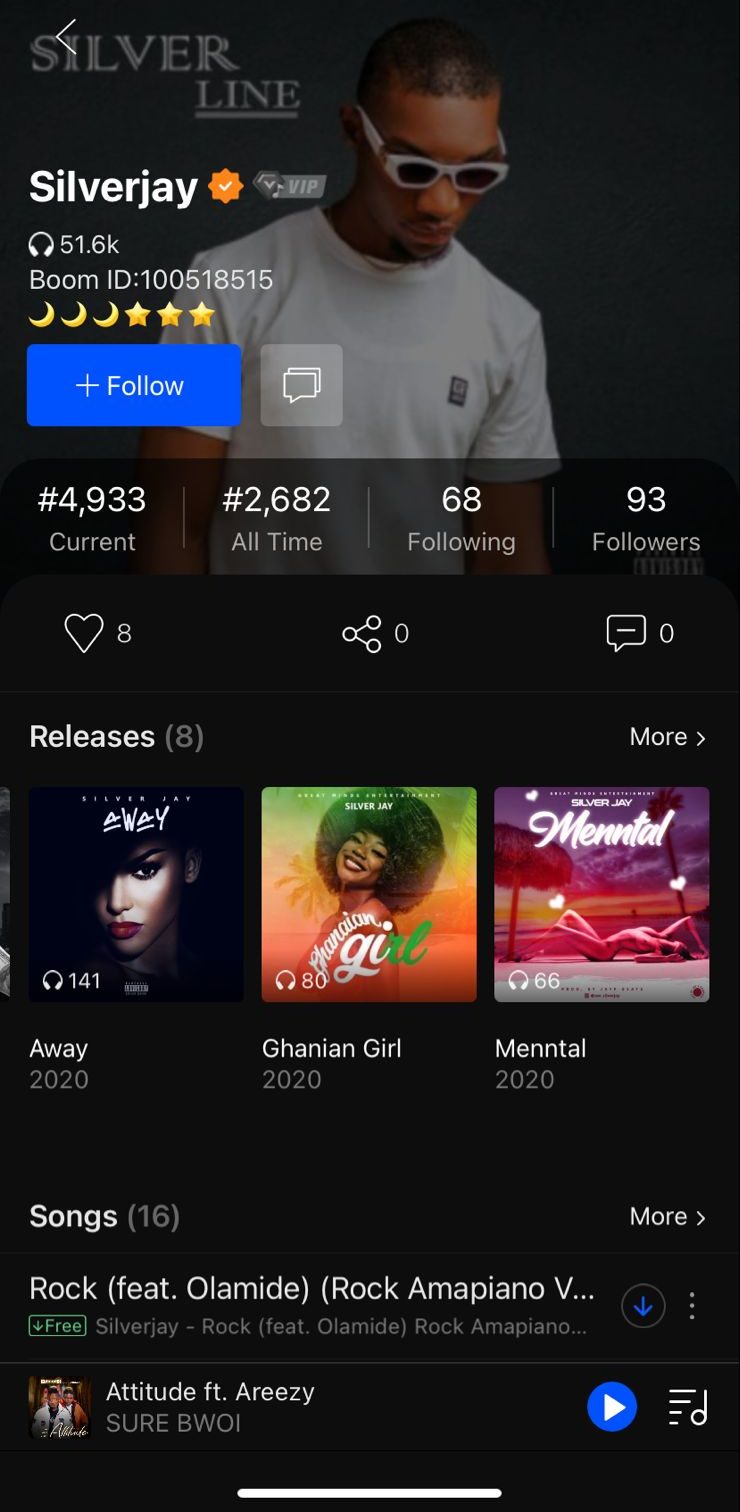The image depicts a comprehensive music streaming app interface. The backdrop transitions from black at the top to various colors as it progresses downward. 

At the top left corner, a white left-pointing arrow is present, accompanied by a notation in silver reading "J". Adjacent to this symbol is an orange circle with a squiggly design that encompasses a white checkmark. Below, white headphones icon prominently displays "51.6K". Below this is text reading "Boom ID 100518518".

Next, there's an icon depicting three yellow moons and three yellow stars. A blue rectangle featuring a white plus sign accompanied by the word "Follow" is also present. A gray square comprised of text boxes follows.

Towards the middle of the image, a man with brown skin and white glasses is seen looking down. He is wearing a white t-shirt. Near him, in white text, several statistics are listed: "#933 current", "#2,682 all time", "68 following", "93 followers", and "8 hearts". 

Additional details include the figure "8 releases," with the term "Away 2020" mentioned. There are also references to "GHANIAN 2020" and "MENTAL 2020". Further, "Songs (16)" is displayed, and it mentions "Rock featuring Olamide," "Olamide rock on my piano," and "Silver J rock featuring Olamide rock on my piano".

Overall, the image provides a detailed snapshot of a music app featuring user stats, engagement icons, and details pertaining to specific songs and releases.